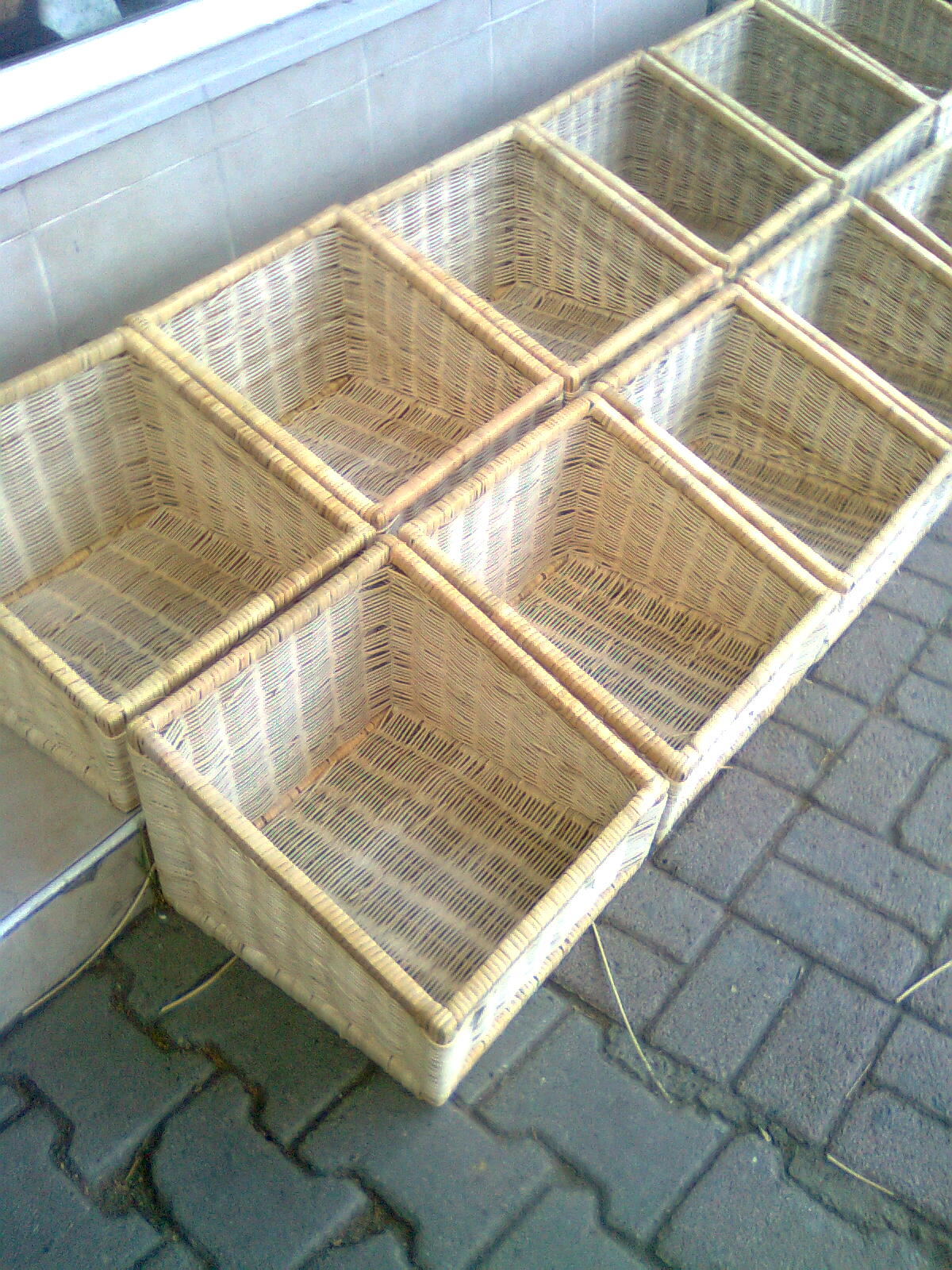The photograph captures an outdoor scene featuring a collection of ten empty, square-shaped woven reed baskets, arranged neatly on a dark brick pavement against a gray cinder block wall. Each basket, a light tan or creamy off-white in color, shows a distinctive design with a lower front and a taller back, creating a seamless, sloped appearance when lined up. These baskets are organized into two rows of five, with the back row elevated on a stepped ledge, enhancing the continuous sloped effect. Small bits of straw are scattered around the bottom left basket, and the backdrop includes a black brick wall and a partial view of a white windowsill, suggesting the location might be outside a business.